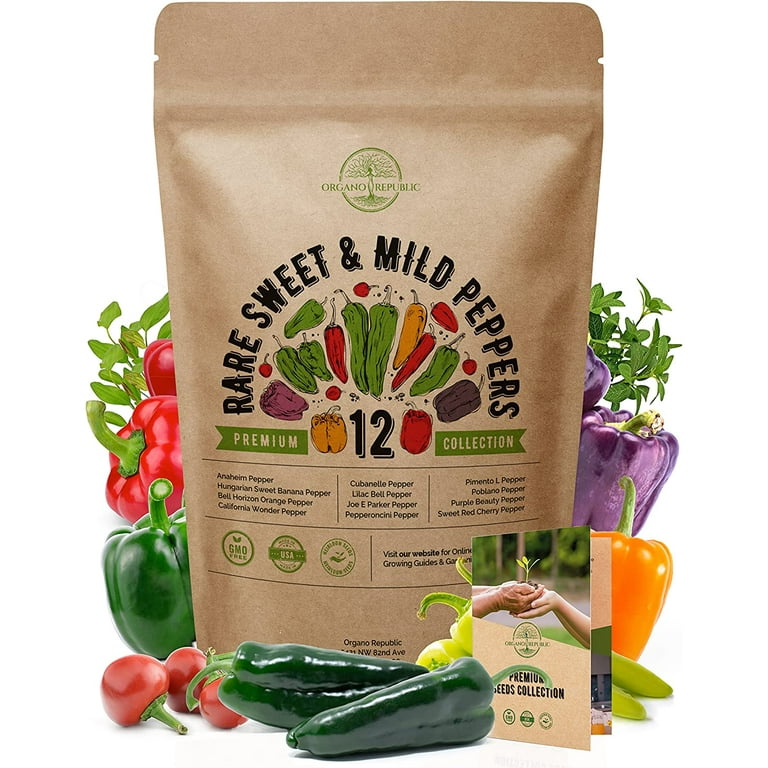The image showcases a sealed brown bag of pepper seeds from "Organo Republic," prominently centered and labeled with "Rare Sweet and Mild Peppers Premium 12 Collection." The bag features a green circle logo with a depiction of a woman rooted to the ground and sprouting branches. Surrounding the bag are various types of peppers in vibrant colors, including red, green, yellow, orange, and purple. Notable peppers visible include red cherry peppers, green jalapenos, anaheim peppers, banana peppers, lilac bell peppers, and poblano peppers. In front of the bag lies a small card titled "Premium Seeds Collection," depicting two hands holding a small sprouting plant. The middle section of the bag illustrates tiny drawings of different pepper varieties listed as part of the collection: Anaheim pepper, Hungarian sweet banana pepper, Bell Horizon orange pepper, California wonder pepper, Cuban L pepper, lilac bell pepper, Joey Parker pepper, pepperoncini pepper, pimento L pepper, poblano pepper, purple beauty pepper, and sweet red cherry pepper. The green circle on the bag also mentions "GMO free, USA," with additional details partially obscured.